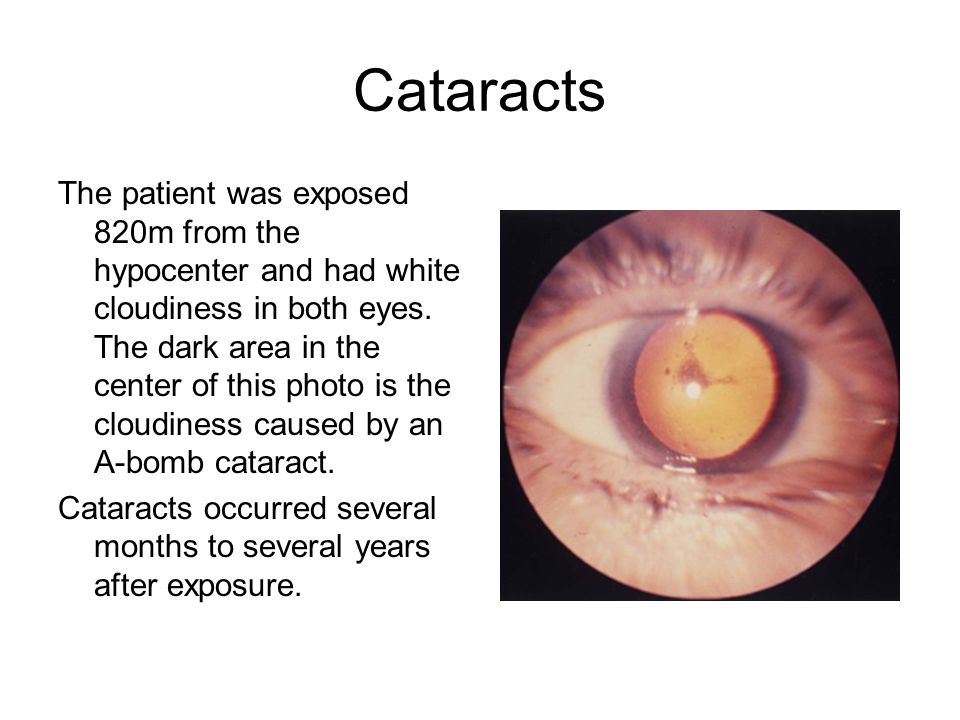This image serves as an educational slide with a white background, prominently displaying the word "Cataracts" at the top in large black letters. The layout is divided into two columns. On the left side, black printed text reads: "The patient was exposed 820 meters from the hypocenter and had white cloudiness in both eyes. The dark area in the center of this photo is the cloudiness caused by an A-bomb cataract. Cataracts occurred several months to several years after exposure."

To the right, there's a square image showcasing a close-up of a human eyeball. The eyeball occupies a circular space within the square frame, focusing on the center of the eye. The eye itself appears predominantly cloudy white, with a golden center and a particular brown fleck. Visible are some subtle flesh tones from the eyelids above and a few eyelashes below. The photograph highlights the characteristic cloudiness associated with an A-bomb cataract, making the condition's visual impact apparent.